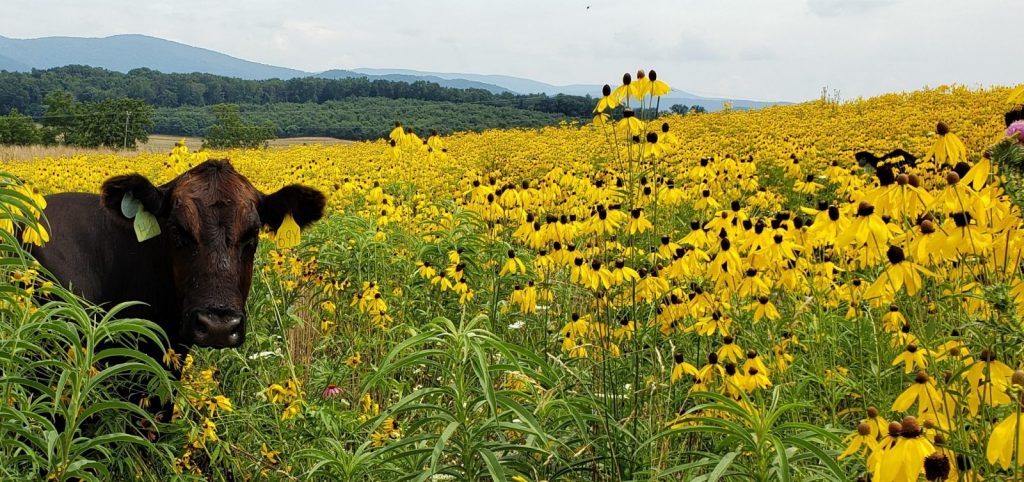In this detailed photographic landscape image, taken outdoors during the daytime, a dark brown cow stands prominently in the left-hand section of the frame, gazing directly into the camera with wide ears and a small green tag dangling from its right ear. The foreground is dominated by a dense area of vibrant yellow flowers with dark brown centers, their petals gracefully tilting downward. These flowers stretch from the bottom right corner and extend upwards towards the middle of the image, interspersed with tall blades of green grass. The middle section showcases a sweeping band of the same yellow flowers spreading across the scene from left to right. In the background, a line of lush green trees transitions into rolling green hills, and further in the distance, a majestic blue mountain range can be seen beneath a light gray, cloudy sky. The composition beautifully captures the serene and vibrant essence of the natural setting.